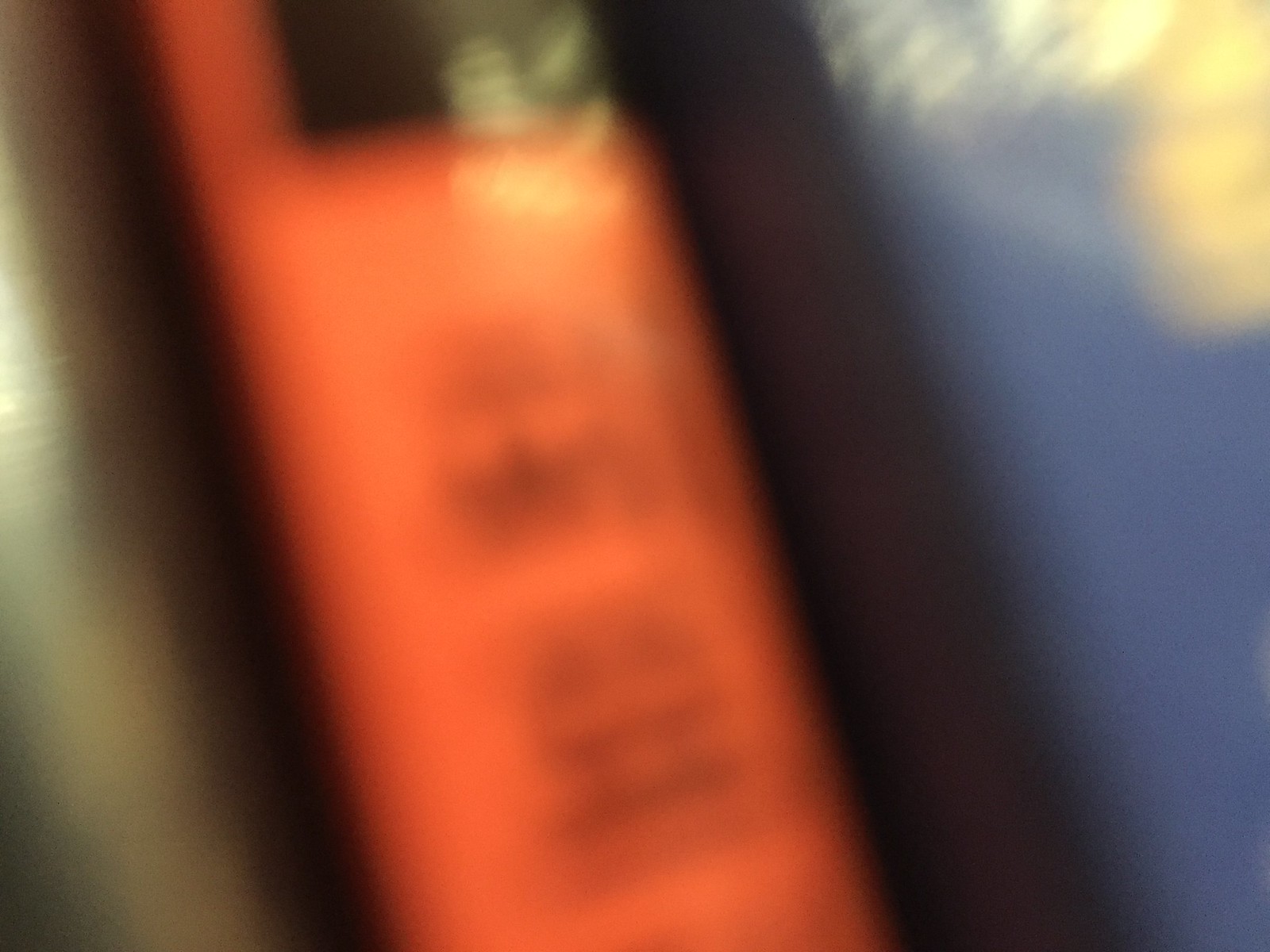This photograph is an extremely blurry image, making it challenging to discern specific details. The most distinguishable element is an orange, bright-colored area positioned at an angle in the center-left of the image, which features some black stripes. This section somewhat resembles the shape of an old phone or could potentially be part of a wall background. The far-right side of the image shows a blue section that appears to be another portion of a wall. The entire left side of the image is dominated by a glare or light, further obscuring the view. The overall scene remains ambiguous due to the high level of blurriness, leaving the exact content of the image open to interpretation.